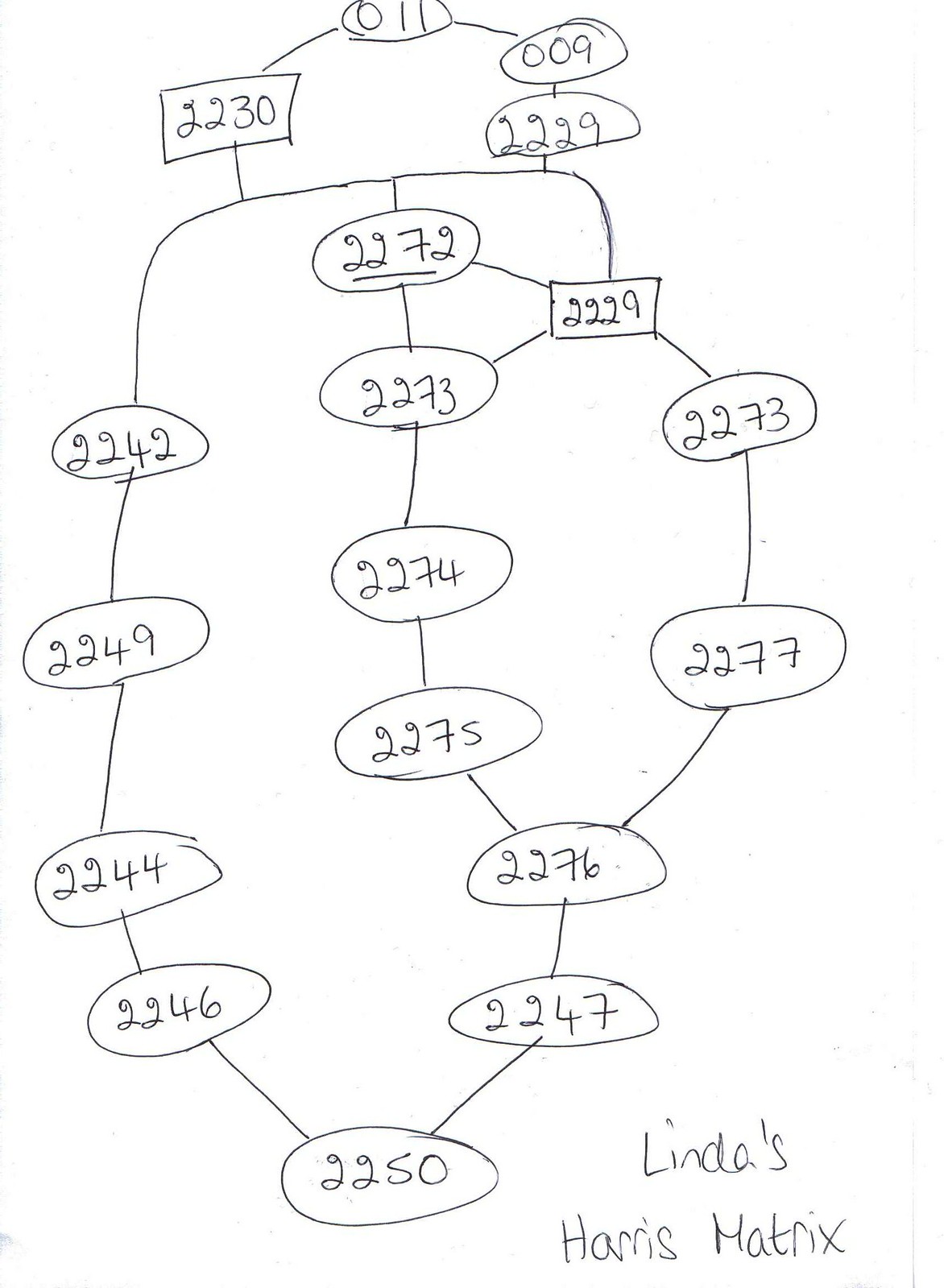The image depicts a detailed Harris matrix, commonly employed in archaeological analysis to illustrate the stratigraphic sequence of an excavation site. The matrix is composed of several numbers enclosed within either oval or rectangular boxes, signifying distinct archaeological contexts or units. These numbers are interconnected by a network of lines, effectively creating a flow graph that extends from the top to the bottom of the image.

At the top of the matrix, the number "011" is prominently displayed, signifying a primary or initial context. This number branches out into two distinct pathways: to the left, it connects to "2230," while to the right, it leads to "009." The right branch further extends downward, creating a loop that includes the number "2229." 

The matrix continues with numerous other connected numbers, ultimately concluding with "2250" at the bottom, indicating the final context in the sequence. In addition, the lower right-hand corner of the image contains handwritten notation that reads "Lender's Harris matrix," identifying it as belonging to a specific project or individual named Lender. The Harris matrix, an essential tool in archaeology, visually represents the chronological order of deposition and stratigraphy, providing critical insights into the temporal and spatial dynamics of the excavated site.